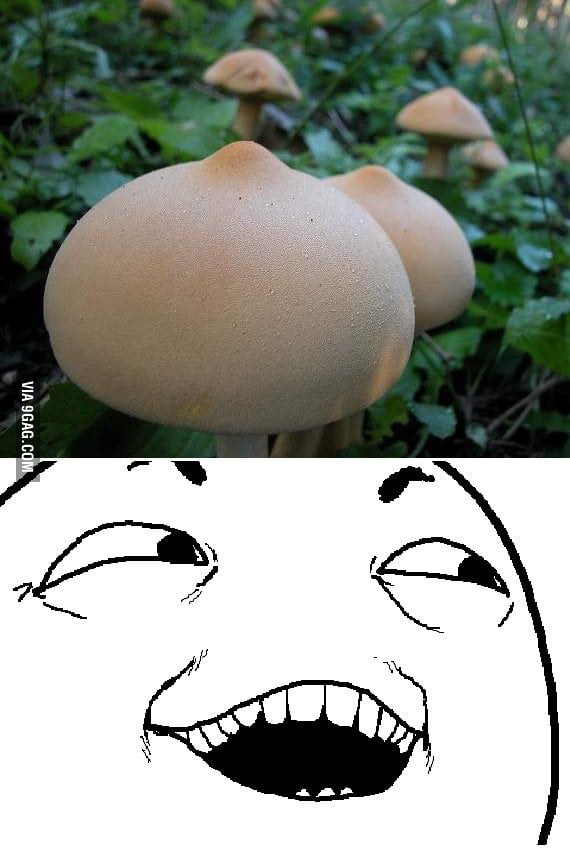The top portion of the image is a detailed photograph of several brown mushrooms with pure brown caps and necks, growing amidst a leafy green setting, indicative of a forest or natural environment. There is a particularly large mushroom in the foreground, with several smaller mushrooms clustered behind it. The overall appearance of the mushrooms is soft and rounded with slightly darker tips resembling domes. Below this photograph is a black and white computer-generated drawing of a cartoonish baby face, characterized by big white eyes, short eyebrows, and a wide smile displaying teeth. A watermark rotated 90 degrees clockwise, from via9gag.com, spans the left side of the image. Additionally, there is another drawing of a stick figure with an open-mouthed, evil grin side-eyeing to the right, adding to the whimsical nature of the composition. The entire image combines natural photographic elements with simplistic, humorous drawings to create an intriguing, multi-faceted visual.